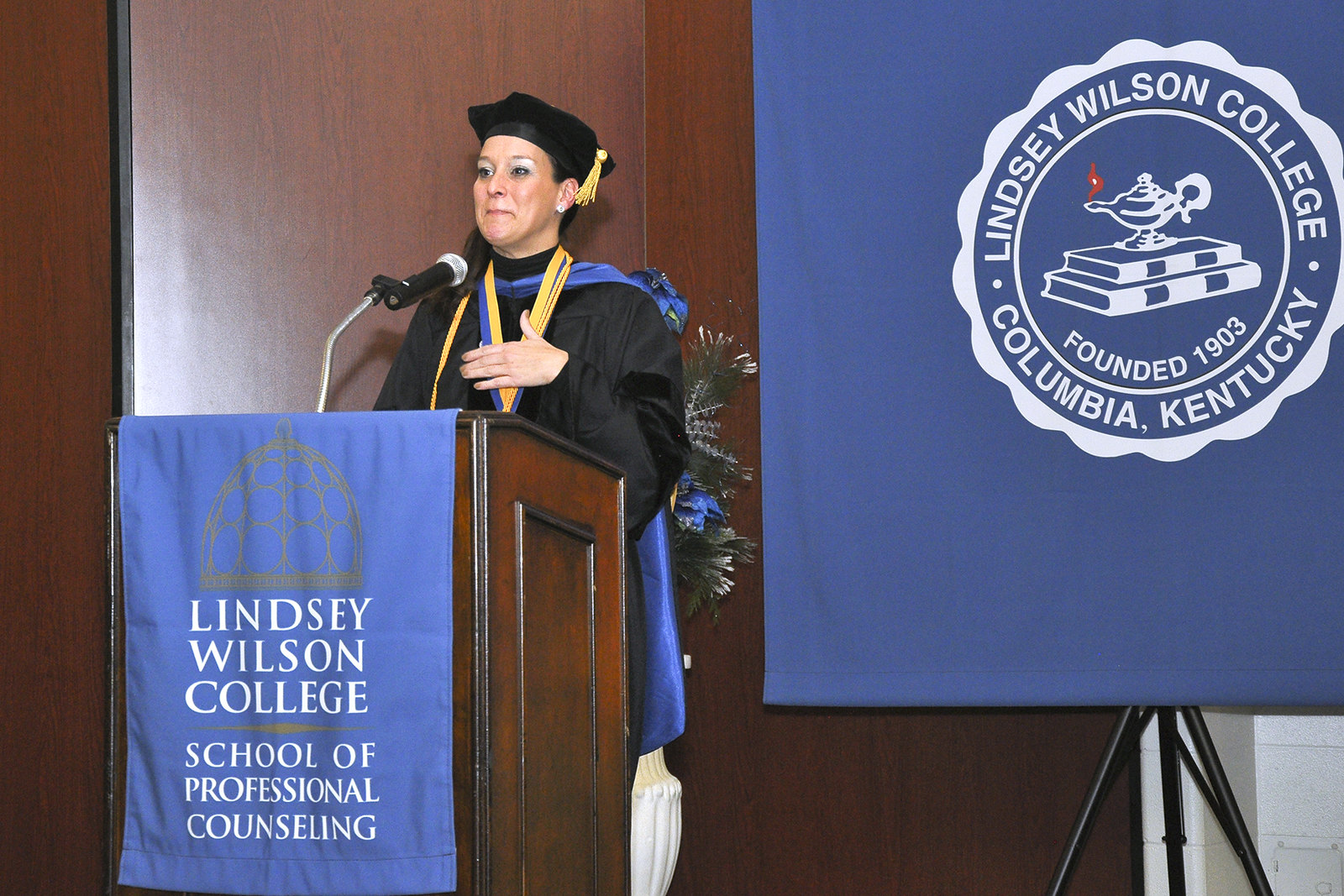The image depicts a woman delivering a speech at a graduation ceremony. She is dressed in a black cap and gown with a gold tassel, and a ribbon with blue and yellow colors around her neck. She stands behind a wooden podium embellished with a blue banner that reads "Lindsey Wilson College, School of Professional Counseling" in white lettering. A microphone is positioned atop the podium. In the background, to her right, there is a tripod supporting a large blue backdrop featuring a circular seal. This seal reads "Lindsey Wilson College, Columbia, Kentucky" with an image of a lamp atop two books in the center and the year "Founded 1903" inscribed below. The setting includes a wood-paneled wall and white concrete or brick surfaces, signifying an auditorium environment. Visible from behind her right side is a partial view of a plant.